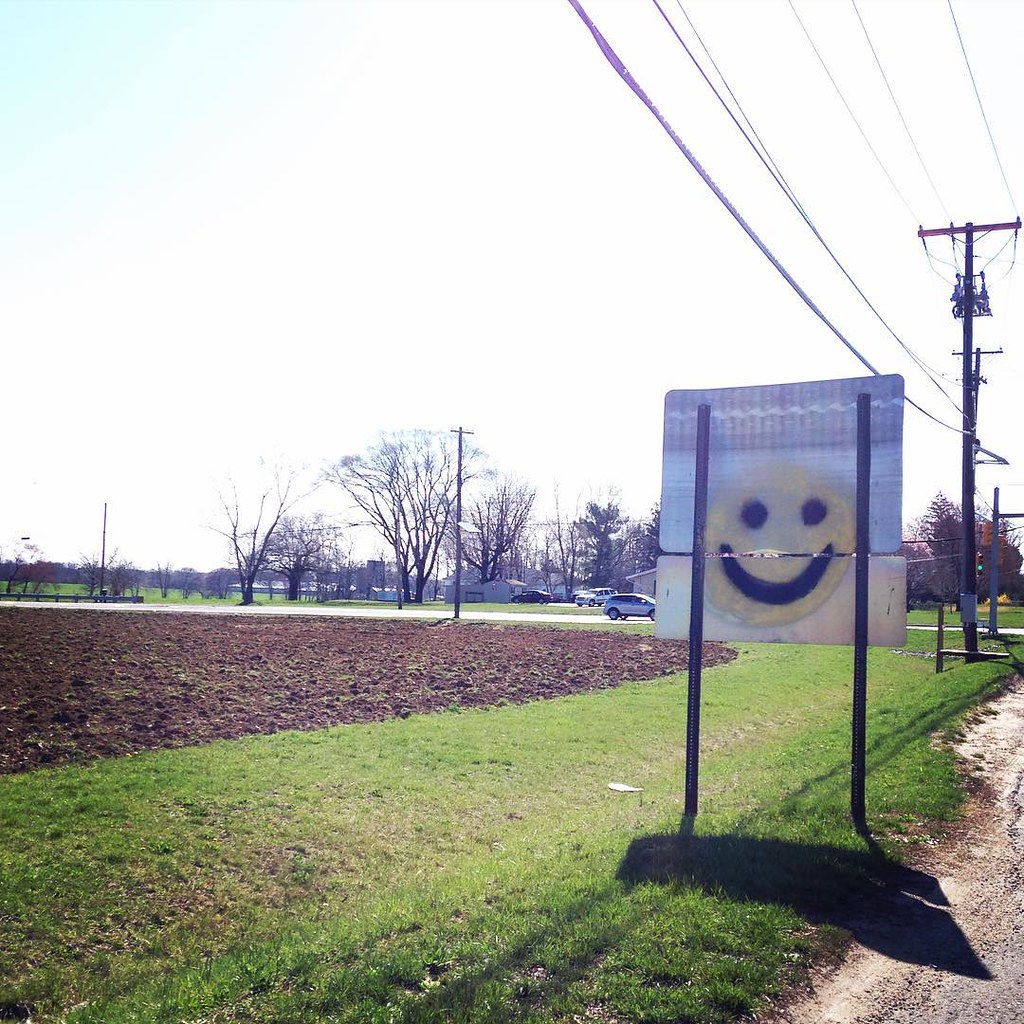In this daytime image taken from the side of a rural road, we see the back of a street sign, which has been spray-painted with a large, yellow smiley face featuring two black eyes and a broad black smile. The smiley face graffiti stands out against the sign's metallic surface. The road is bordered by a strip of grass with patches of brown, suggesting dryness. Adjacent to the grass is a large dirt field, possibly prepared for crop planting. The scene appears to be set in late fall or winter, as the trees in the background are devoid of leaves. The sky is primarily a pale blue that fades into a white, and it casts clear shadows from the street sign, telephone poles, and power lines onto the ground. In the distant background, there are several houses and parked cars, with more greenery and flat terrain stretching out. A green traffic light is visible in the upper right corner, along with some moving vehicles on the road.